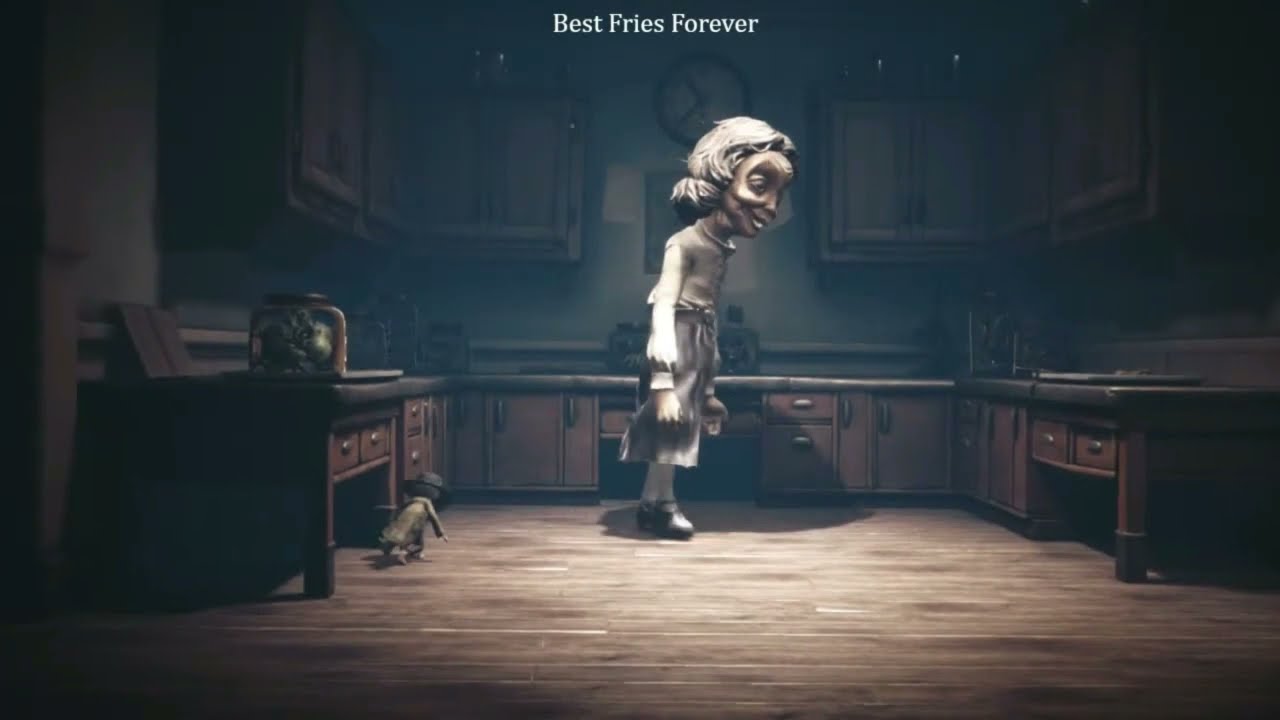The image depicts a dark, dimly-lit kitchen with only a single overhead light illuminating a central figure and casting shadows around the edges. Central to the composition is a caricature of an old woman with a weary, sad expression and hanging head, emphasizing her dejected demeanor. She wears a white dress with a high collar, long sleeves, an apron, tights, and grayish metallic shoes. Her hair is gray and cut short. The exaggerated scale of the background elements, like the low countertops and raised-legged table, give her an unusually imposing height, adding to the surreal atmosphere. To her left, partially obscured, crouches a small child-like figure—or possibly a monkey in a yellowish-brown dress, with black hair. The child appears to be sneaking behind her. Above the scene, the text "Best Fries Forever" is displayed, while the kitchen, with its dark cabinets and wooden floor, has a clock mounted over the sink. Overall, the setting and characters create a hauntingly detailed, almost eerie depiction of domestic life.